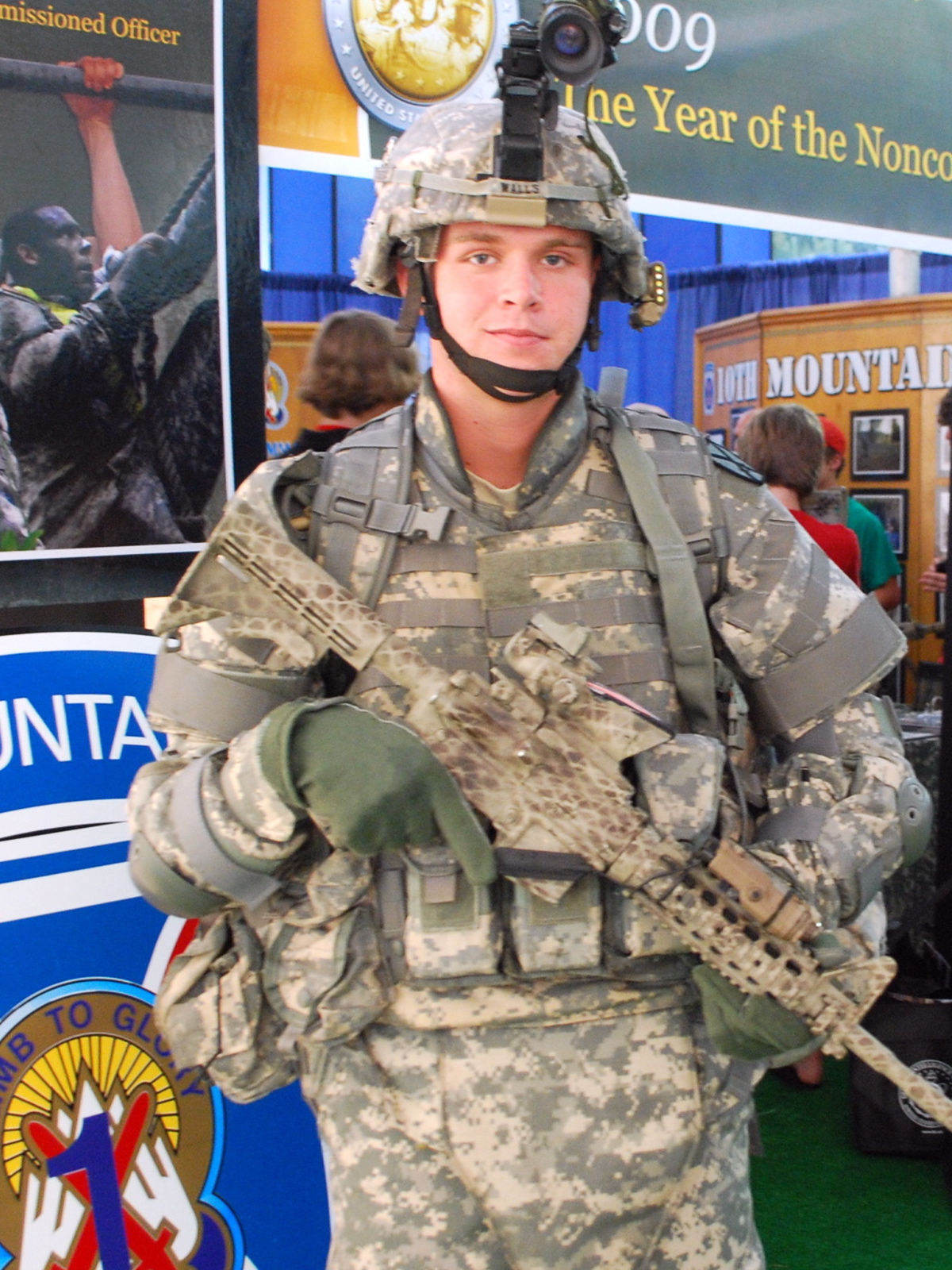The photograph captures a soldier in a standing position, showcasing his face and upper body. He is fully dressed in a grey and cream-colored uniform, including a helmet fitted with a mounted camera and a chin strap. The soldier carries a cream and brown camouflage rifle, and additional gear adorns his attire, including a backpack, several pouches, and bags hanging from his waist belt. In the background, various elements are visible, such as posters, an identifiable display referencing the "10th Mountain" division, and a partially obscured blue logo. A person holding a microphone appears in the upper left corner, and another individual is seen in what may be a booth area. The scene suggests a recruitment or public display setting, possibly at an event highlighting different career opportunities like those found in a college recruitment fair. The soldier's helmet also bears what appears to be his last name, "Walls," and an unclear inscription related to his rank or unit.